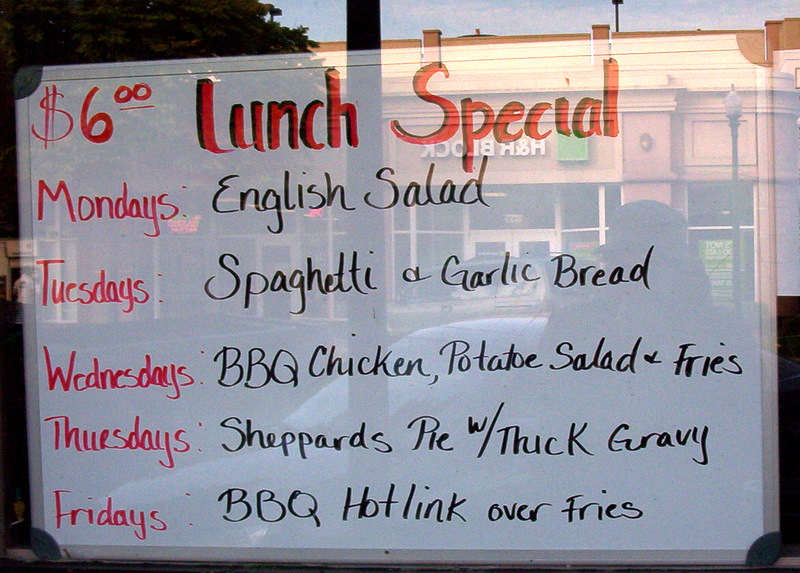The photograph captures a large whiteboard sign placed behind a window, likely of a restaurant, indicating the weekly lunch specials. The sign prominently displays "$6 Lunch Special" written in red, with "Lunch Special" also featuring a black shadow script. The menu is organized with the days of the week listed on the left in red, and the corresponding specials on the right in black marker. Specifically, the menu includes:

- Mondays: English Salad
- Tuesdays: Spaghetti and Garlic Bread
- Wednesdays: BBQ Chicken, Potato Salad, and Fries
- Thursdays: Shepherd's Pie with Thick Gravy
- Fridays: BBQ Hot Link over Fries

The whiteboard itself has black attachments at the corners. Reflected in the window, the storefront of an H&R Block is visible, as well as a person looking at the menu and a parked car, indicating it is daytime.